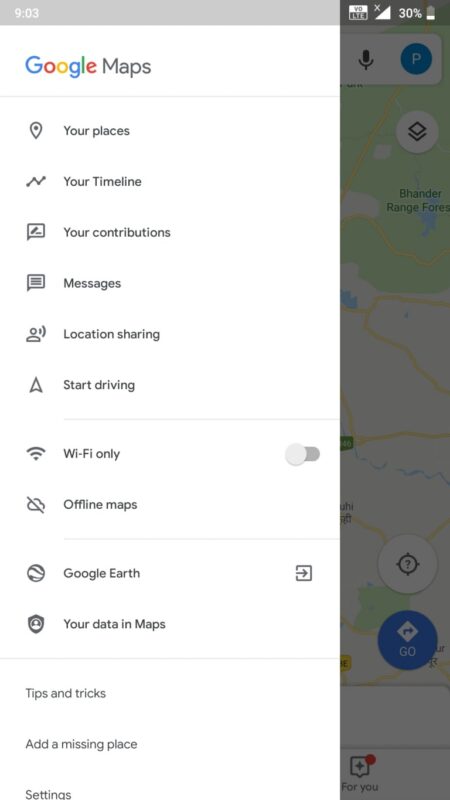The image displays a mobile device screen with a white background. At the top-left corner, the screen shows "30% battery" and the current time as "9:03". Dominating the center of the screen is the iconic Google logo, featuring letters in a variety of colors: two blue G's, a red O, a yellow O, a green L, and a red E, with a line underneath it.

Below the logo, a list of features is presented, each accompanied by a distinctive icon to its left:

- "Your Places" - symbolized by a red location pin.
- "Your Timeline" - denoted by a clock face.
- "Your Contributions" - represented by a star.
- "Messages" - marked with a blue speech bubble icon.
- "Location Sharing" - indicated by two overlapping circles.
- "Start Driving" - signified by a car icon.
- "Wi-Fi Only" - displayed with a Wi-Fi symbol.
- "Offline Maps" - depicted with a downward arrow on a map.
- "Google Earth" - indicated by a globe icon.
- "Your Data in Maps" - shown with a shield icon.
- "Tips and Tricks" - illustrated with a light bulb.
- "Add a Missing Place" - denoted by a plus sign in a circle.
- "Send Feedback" - represented by an exclamation mark in a speech bubble.